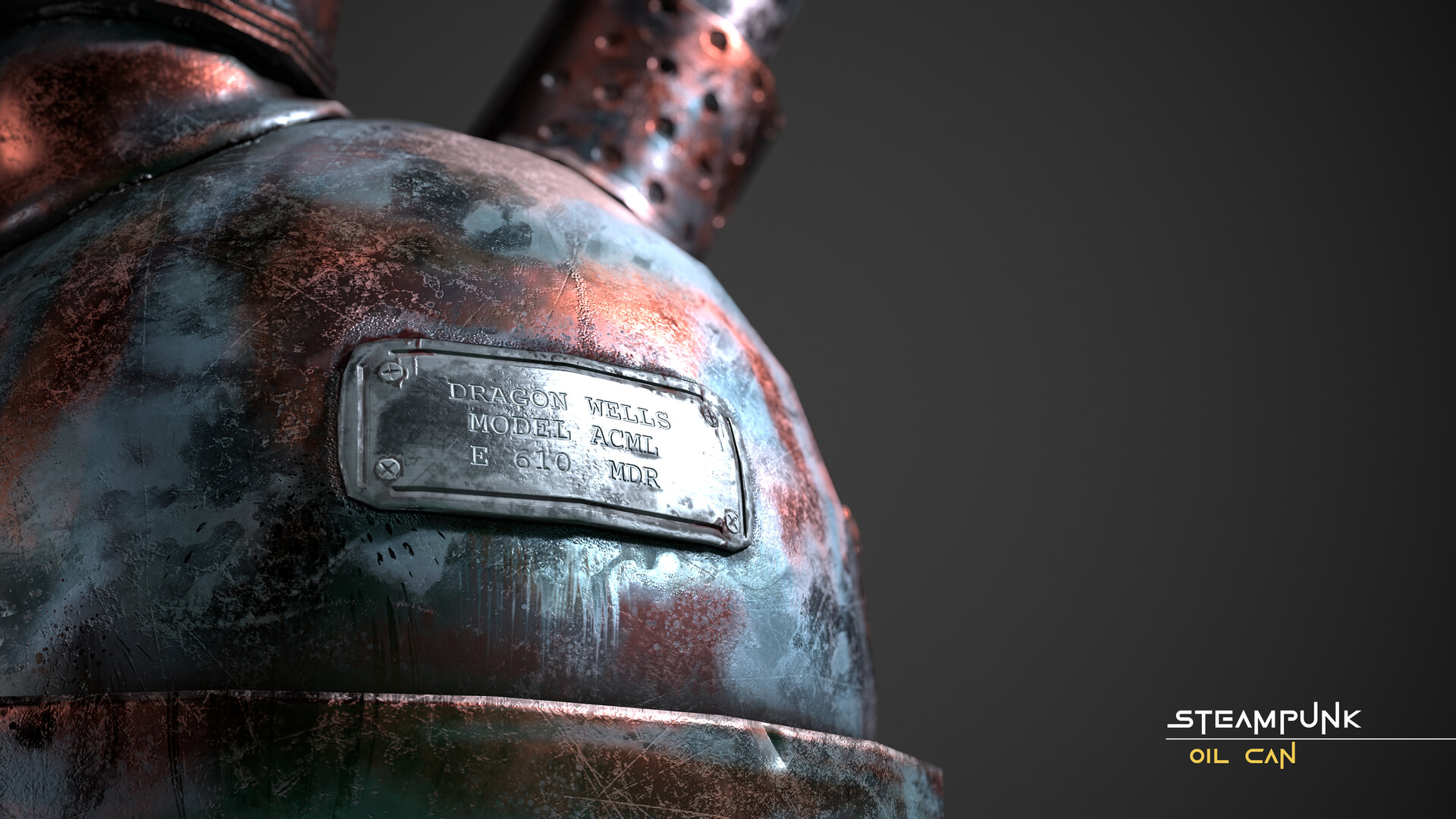The image depicts a vintage Steampunk Oil Can with a patina of age, set against a gradient gray background that darkens toward the edges. The oil can, primarily made of metal, features a faded copper hue interspersed with silver tones, indicative of corrosion over time. The can's design is intricate, having a dome-shaped top with two extensions resembling spouts. One extension appears to be where the oil is dispensed, decorated with various holes, while the other might be a screw-off cap for oil refills. A metallic nameplate is prominently affixed with screws, displaying the inscription "Dragon Wells Model ACML E610MDR." This label, along with the overall metallic gleam and the Steampunk aesthetic, underscores the can's antique charm. The words "Steampunk Oil Can" are visible at the bottom right corner of the image.